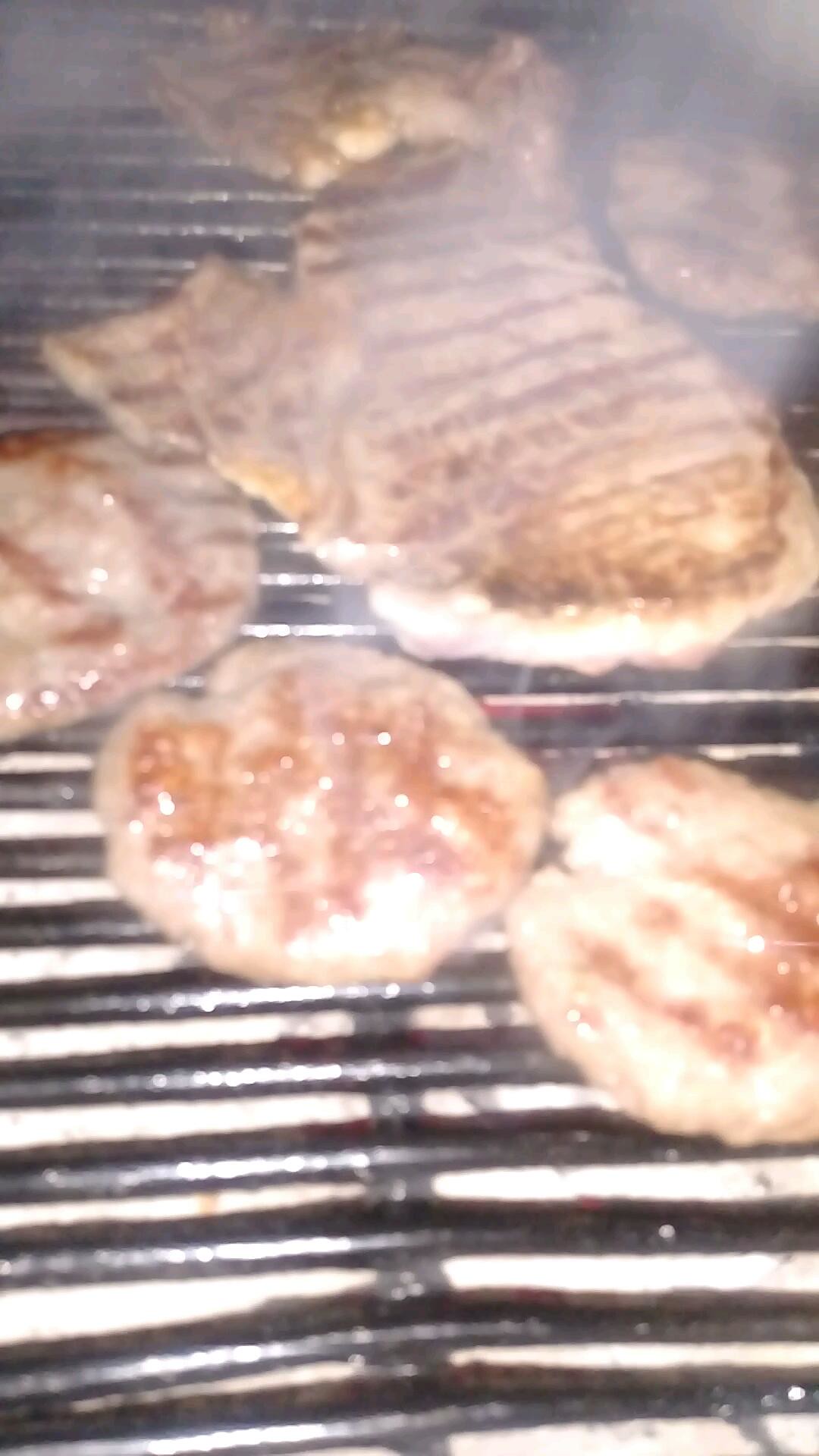In this out-of-focus, blurred color photograph taken in portrait mode, an assortment of meat is grilling amidst light gray smoke. The black metal horizontal bars of the barbecue grill are visible through the haze of steam. In the foreground, three round burger patties with distinct grill marks sit alongside a larger, irregularly shaped flat steak. Another round piece of meat with similar grill marks is visible in the background on the right. The meats are light brown with no visible pink or blood, and the photo captures the scene from a slanted angle without any visible flames.